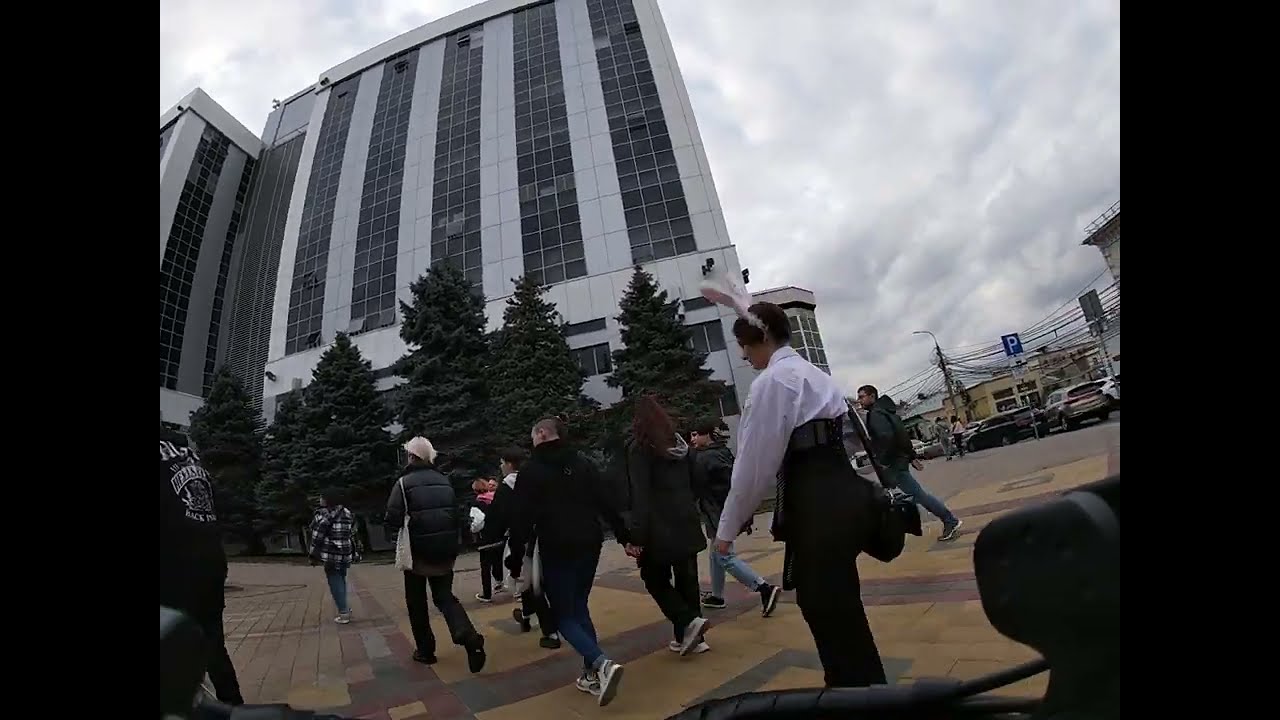This daytime outdoor photo captures an overcast atmosphere with a touch of whimsy, set against the backdrop of a tall, wide white building featuring distinctive black grid-patterned windows. In the foreground, a diverse group of pedestrians crosses a patterned stone walkway, adorned with hues of yellow, red, and green. A noteworthy figure in the scene is a woman on the far right, drawing attention with her white bunny ears, white long-sleeve shirt, black corset, and black slacks, adding an unexpected twist to the otherwise mundane moment. Surrounding the building are several pine trees, electric poles, parked cars, and a parking sign. The overall scene is bustling yet grounded by the solidity of the architecture and the natural elements interspersed throughout.